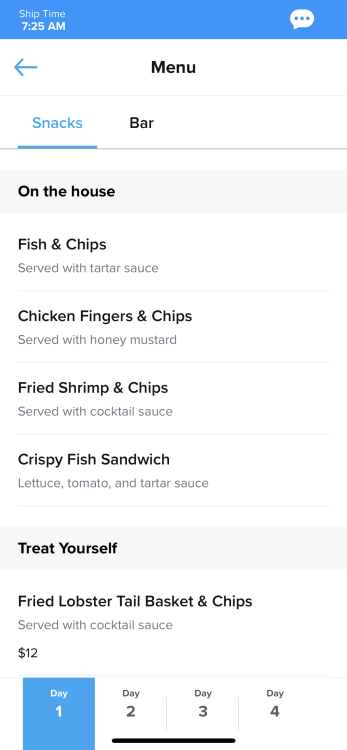The image is a screenshot of a cell phone screen displaying a food menu interface. The screenshot has a vertical orientation. The background is predominantly white, slightly distinguishable from the cell phone screen's bordered background. 

At the top, there is a blue banner with white text. In the upper-left corner, it states "Ship Time: 7:25 a.m." On the upper-right corner, there's a comment bubble icon with three dots inside it, indicating additional options. Centered below the banner is the word "Menu," accompanied by a blue arrow pointing to the left, suggesting a back navigation function.

Beneath the "Menu" heading, users can toggle between "Snacks" and "Bars," with "Snacks" currently selected and underlined in blue. The selected menu category features a list of food items with black text for the entree names and gray text for their descriptions.

The list of options includes:
- Fish and Chips: Served with tartar sauce.
- Chicken Fingers and Chips: Served with honey mustard.
- Fried Shrimp and Chips: Served with cocktail sauce.
- Crispy Fish Sandwich: Includes lettuce, tomato, and tartar sauce.

There is also a "Treat Yourself" section offering a special dish:
- Fried Lobster Tail Basket and Chips: Served with cocktail sauce, priced at $12.

Other items in the list do not display prices, indicating they may be standard menu options. There might be additional menu entries that would require scrolling down to view.

At the bottom of the screen, there is a navigation bar with four options labeled "Day 1," "Day 2," "Day 3," and "Day 4." "Day 1" is highlighted with a blue box around it, suggesting that it is the currently selected day or menu.